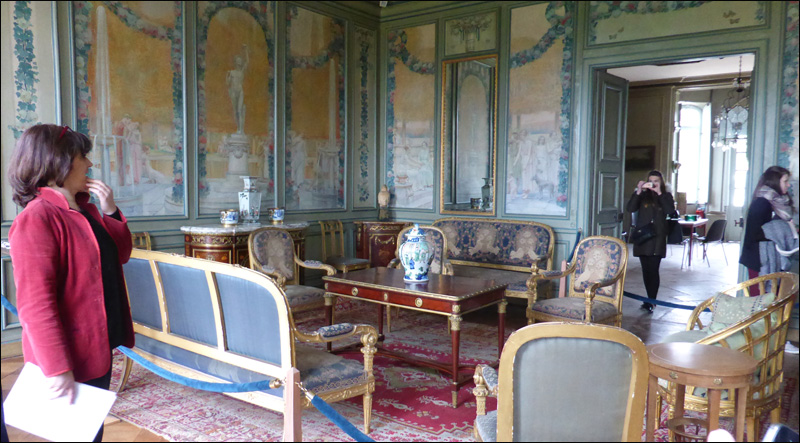The photograph captures a palatial room in a historical building, teeming with opulent furniture and artwork. The room is lit by natural daylight streaming through a large window in the far upper right corner, enhancing the room's intricate details. Dominating the center, a large red-stained table holds a striking white and blue urn. Surrounding the table are multiple chairs, arranged meticulously. Two blue-and-gold patterned benches, resembling couches with armrests, and matching armchairs flank one side of the room. On the opposite side, two distinct armchairs with green cushions and gold-painted wood frames add to the intricate decor.

The walls are adorned with various artworks, and the entryways are grand and inviting. A beautiful oriental rug graces the floor, adding to the rich visual tapestry. Above, an unlit chandelier hangs majestically. Velvet ropes cordon off sections of the room to preserve the pristine condition of the antique furniture. 

Three people are visible in the image: a woman in a red jacket stands close to the left, another woman is seen in the back taking a picture, and a third woman walks away, indicating the room's current use as a tourist attraction. The colors throughout the room range from whites and light blues to eggshell, reds, pinks, purples, and various shades of brown and blue, creating a harmonious and elegant palette typical of a grand, historic setting.